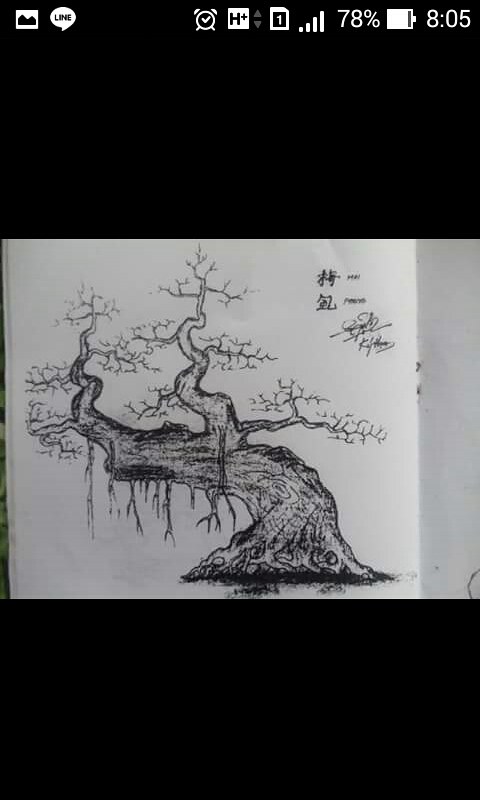This image appears to be a photograph taken with a phone, showcasing a pencil sketch of a tree, possibly a bonsai, that strongly conveys Japanese influences. The sketch, set against a black background, is intricate and detailed, featuring a tree with a main trunk that bends distinctly to the right, from which several branches extend both upwards and to the sides, resembling the delicate, flowing lines of a weeping willow. The bonsai tree stands prominently in the center of the drawing, with fine branches that almost look eerie, reminiscent of a tree from a horror movie. On closer inspection, the lower part of the tree's trunk appears to have two small, eye-like shapes, adding to its eerie allure. 

To the left of the bonsai, there are Japanese characters, situating the tree within a cultural context. The digital photo of this drawing is framed by the phone's interface, with black borders on either side and a top bar showing various notifications: the time is 8:05, the battery is at 78%, and it has five signal bars. Multiple notifications, including an alarm and a gallery icon, indicate that the photo is being viewed from a personal gallery, reaffirming its digital origin.